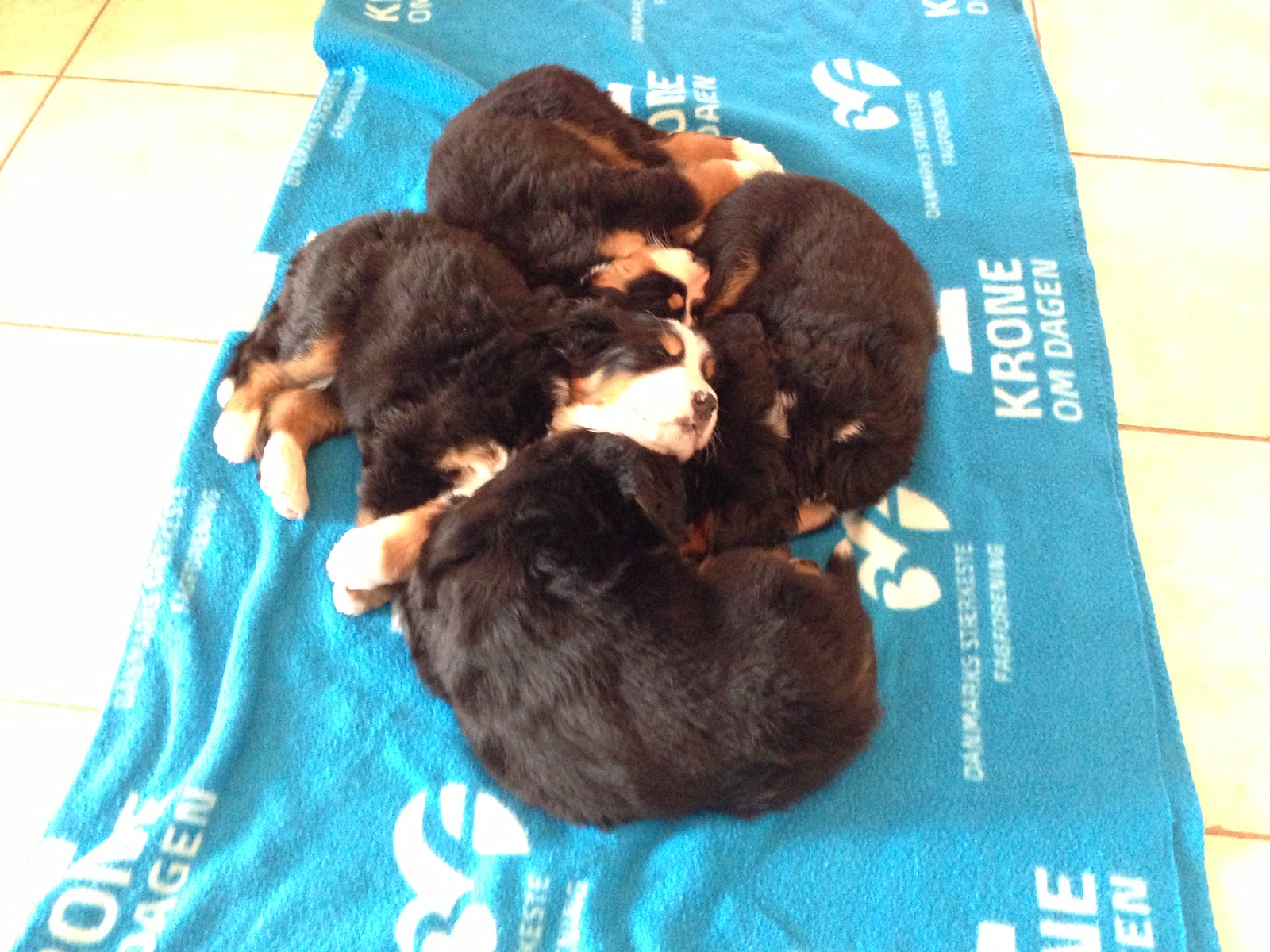The photograph captures a serene moment featuring five small, black puppies with brown legs and white-tipped paws, all cozily sleeping together on a large, light blue beach towel laid out on a cream-colored square tile floor. The puppies exhibit white fur on their muzzles and each has floppy ears, with some of their faces hidden beneath the heads of their siblings. The blue towel, oriented vertically within the image, bears white text spelling out "KRONE OM DAGEN" along with a logo resembling either a number three or paw prints. The peaceful jumble of puppies epitomizes comfort and warmth as they nestle closely, resting on top of one another.